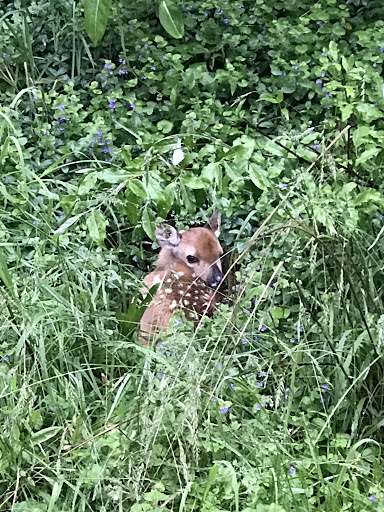In this vibrant outdoor photograph taken on a sunny day, a young fawn is nestled amidst a dense and lush field of tall grasses and various green plants. The fawn, identifiable by its brown fur adorned with white spots reminiscent of Bambi, is draped across the center of the image. Its small body is surrounded by an array of vegetation, including slender leaves, broader leafy shrubs, and interspersed wildflowers, some with hints of blue and purple blossoms.

The scene is teeming with life, showcasing the diversity of plant species from leafy vines to tall, wheat-like grasses. The fawn’s head is turned back, glancing over its shoulder with large black eyes, a black snout, and delicate, pink-lined ears with white fur interiors. The light brown fur on its face contrasts with the darker brown of its back, creating a striking image against the vibrant green background.

Despite being partially concealed by the dense foliage, the fawn’s alertness is palpable, as it stares intently in the direction of the photographer. The overall composition captures the intimate moment of this young deer possibly hiding within the verdant embrace of the overgrown meadow, bathed in natural sunlight reflecting off the myriad leaves.